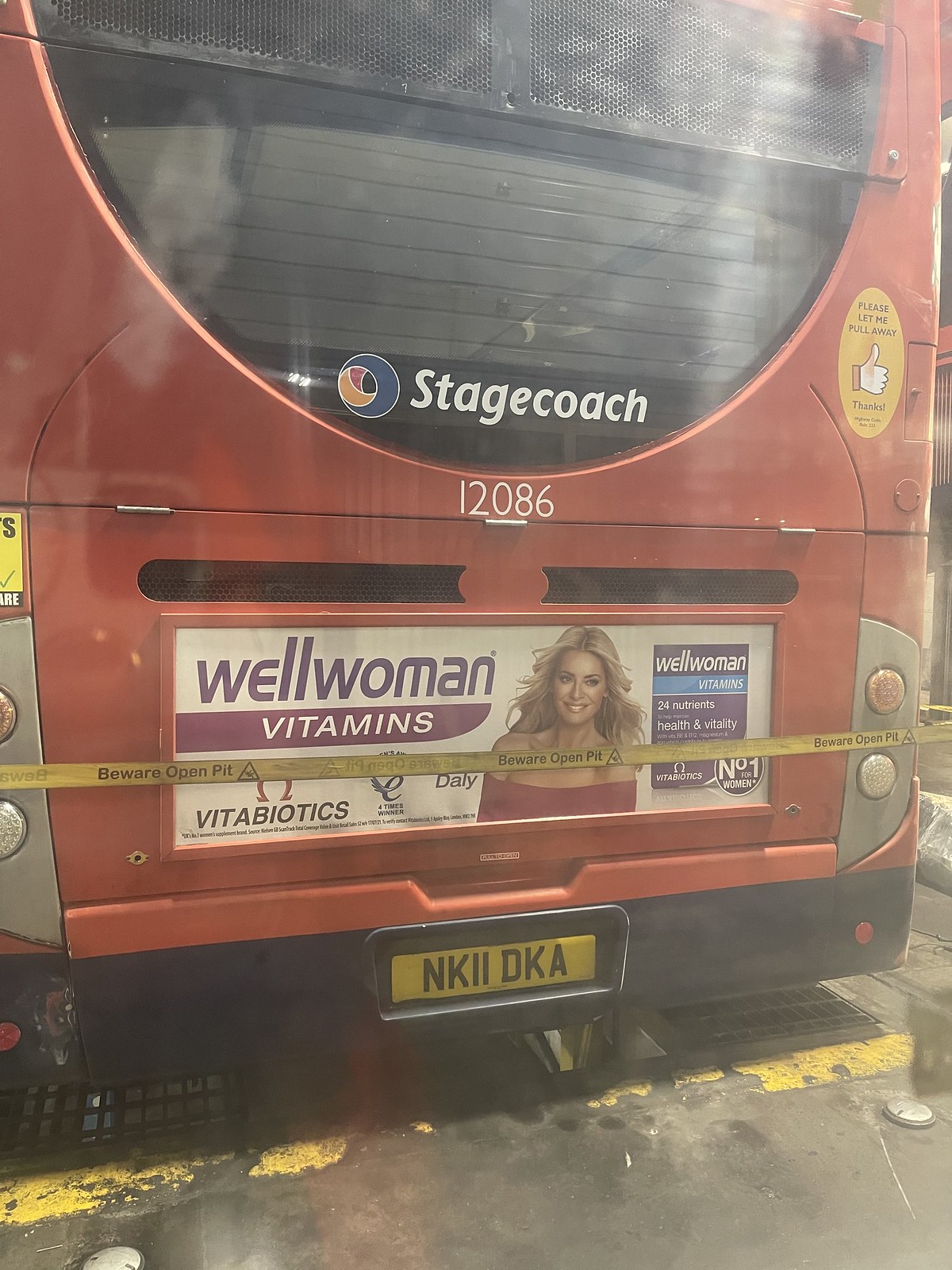The photograph prominently features the back end of a large, foreign-made red-colored bus, identified as a Stagecoach. The bus has a somewhat vintage appearance, with a round window on the back that is covered by blinds. Notably, the bus displays the number 12086 in white lettering. Dominating the central part of the image is an advertisement for Well Woman Vitamins by Vitabiotics, which features a beautiful young lady with long, flowing blonde hair, a bright white smile, and captivating eyes, dressed in an off-the-shoulder red top. The advertisement has a white background with purple lettering, promoting the message "24 nutrients, health and vitality, number one for women."

Below the advertisement, you notice a black bumper adorned with a yellow license plate reading "NKII-DKA" in black lettering. On either side of the advertisement are what appear to be backup lights. The setting appears to be either outdoors or in a garage, as indicated by the concrete surface with yellow lines and a visible curb to the right. Additionally, a yellow caution ribbon around the back of the bus warns of an open pit. Another small sign on the bus reads "Please let me pull away" with a thumbs-up icon, adding a touch of courtesy to the scene.